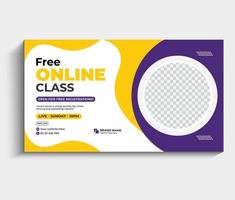The image features a small, colorful business card or postcard set against a bluish-white background. The card is predominantly accented with purple, yellow, and white. On the left side, there is a decorative white square containing the bold black text "FREE," with the word "ONLINE" in larger yellow capital letters just below it. Below "ONLINE," the word "CLASS" is written in smaller black capital letters. 

The right side of the card features a purple section with a distinctive white circle at the center, within which is a smaller circle filled with a grey checkerboard pattern, resembling a scratch-off area. Below this circle, there are additional words in purple and yellow, including a purple bar with text that is too small to be legible, followed by a yellow bar with more text and what appear to be social media handles. The overall layout divides the card into an approximate two-thirds to one-third split, creating a dynamic and eye-catching design emphasizing the offer of a "Free Online Class."